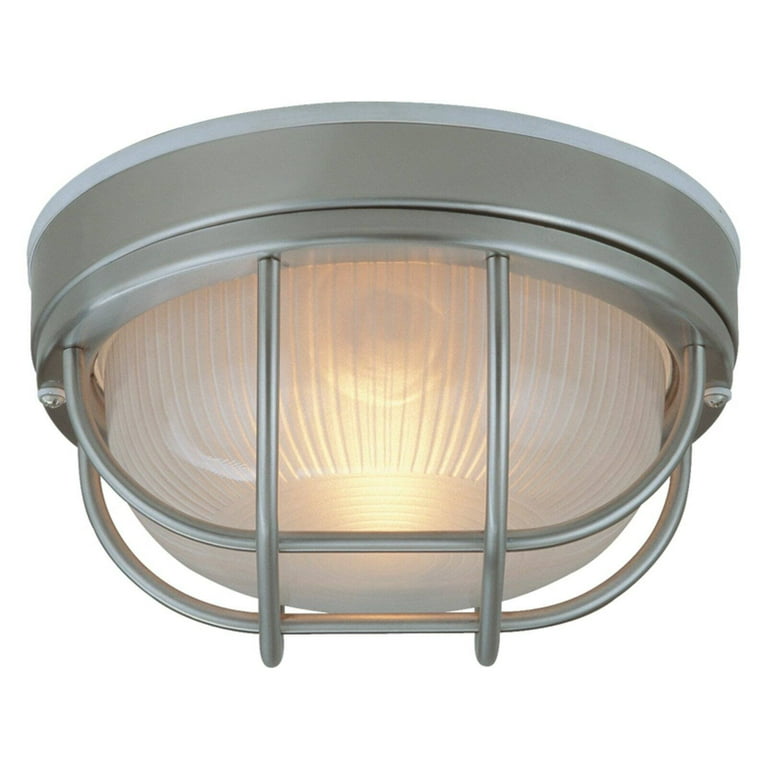The image showcases a gymnasium-style light fixture with a sturdy aluminum and silver exterior. The light itself emanates a soft yellow glow, encased in a somewhat transparent, easily breakable white plastic covering. To protect the fixture from impacts, such as from volleyballs, softballs, or basketballs, there is a robust silver grating around it. This protective grating is sturdy and has a textured, scalloped edge, not perfectly smooth. The exterior also features some black indents on the silver protector, adding to its secure design. There is no additional text, numbers, or other objects in the image, leaving the light fixture as the primary focus.